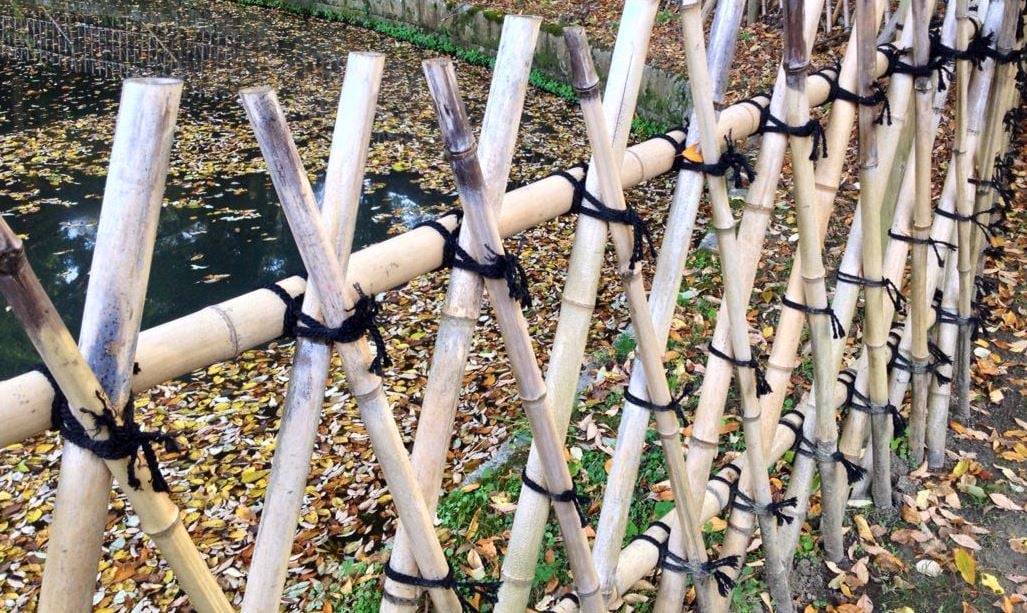This photograph taken outdoors features a meticulously constructed bamboo fence crisscrossed in an X pattern and secured with dark rope. The bamboo, with its yellowish-tan hue, forms a sturdy barrier consisting of two horizontal rows of bamboo, reinforced vertically by crossed pieces that create repeating triangle shapes. Behind this carefully tied fence lies a small, man-made lake or pond, partially contained by a concrete barrier. The water surface is heavily adorned with fallen leaves of various colors—yellow, white, and red. In the bottom right corner, a dirt pathway runs just outside the bamboo fence, adding to the scene's rustic charm. The overall composition suggests a serene, natural environment, accentuated by the intricate craftsmanship of the bamboo fence and the autumnal leaves floating on the tranquil water.